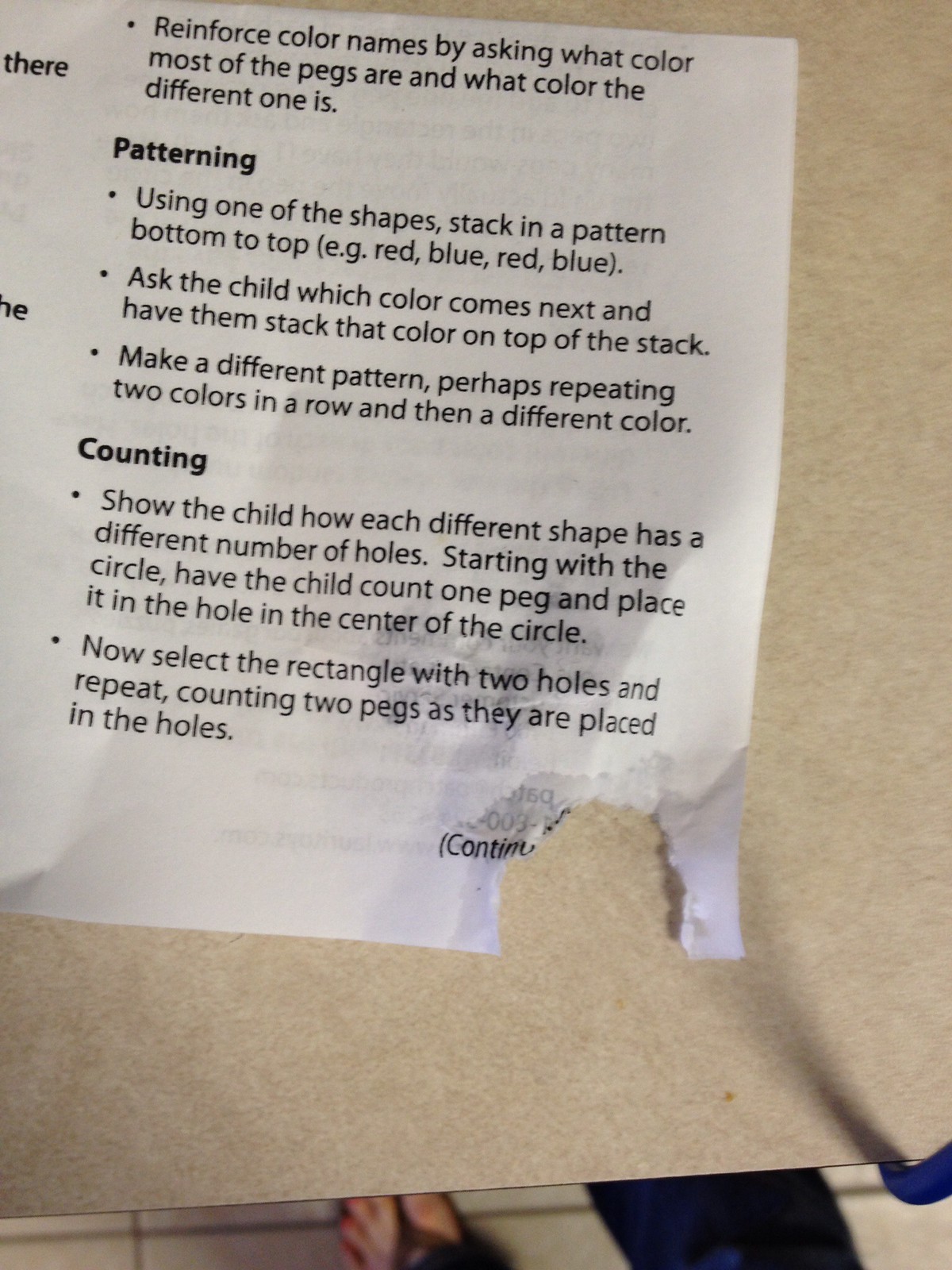A computer-printed instruction sheet, possibly from a book or educational pamphlet, lies on a pebbly gray or tan countertop. The sheet, resembling an 11 by 17 piece of paper, has been partially torn and water-damaged in the lower right corner. The paper is divided into two columns, but the left column is nearly cut off and unreadable. The right column is visible and includes two bold subject headings: "Patterning" and "Counting."

Under "Patterning," the instructions detail using shapes to create color patterns, such as "red, blue, red, blue." Children are prompted to identify and continue the sequence by stacking the appropriate color. The text begins with the directive: "Reinforce color names by asking what color most of the pegs are and what color the different one is."

The "Counting" section focuses on teaching numbers through shape recognition. The instructions guide showing how each shape correlates with a different number of holes, progressively increasing from one to more. For example, starting with a circle containing one hole, the child is asked to place one peg in it, followed by a rectangle with two holes and counting two pegs into it.

In the background of the image, the flip-flop-clad feet of an individual are faintly visible at the bottom, adding a subtle human element to the scene.